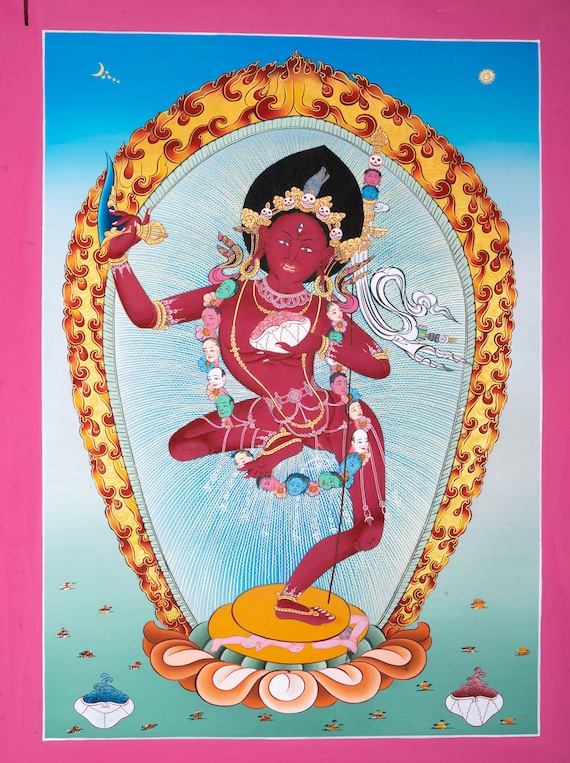The image depicts a striking illustration of a Hindu goddess, depicted with an intense, almost fierce expression. She stands on one foot, balancing gracefully on a lotus flower, and appears to be levitating. The background transitions from blue to white to green, enhancing the ethereal ambiance around her. Her reddish-pink hued figure is adorned with intricate details: a crown decorated with little skulls and gold flowers, topped with what appears to be a snake head. Her hair, styled upward in a point, frames her solemn face, which features a third eye on her forehead. 

Her extended earlobes are adorned with large, heavy-looking gold hoop earrings, and she also wears dangling earrings that complement the garland of little heads draped around her neck. This garland extends down to her feet and around one of her hands. In her left hand, she holds a shell filled with something pink, while her right hand grips an object that appears gold and blue, reminiscent of a lava lamp. Surrounding her are more lotuses and two additional shells—a blue one on the left and a red one on the right. An arc with a small moon on the left and a tiny sun on the right further accentuates her divine presence, while smoke or mist emanates from her ornate headpiece, adding to the mystical and sacred feel of the image.